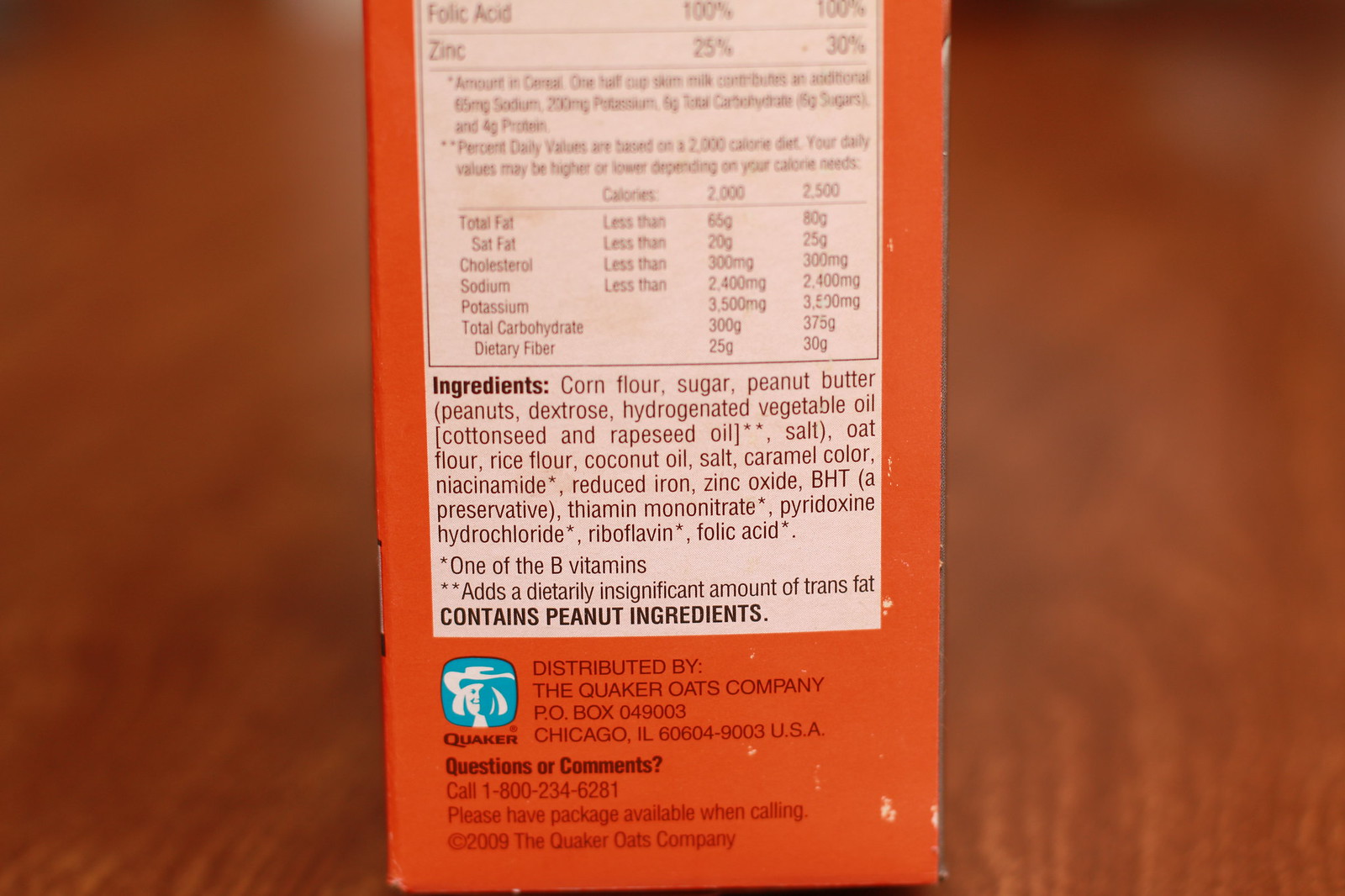The image is a photograph of the side of a cereal box, positioned against a brown wooden surface. The box itself is predominantly red, with a white nutrition label centrally displayed. At the top of the label, the nutritional information highlights key values like folic acid at 100%, zinc ranging between 25-30%, with details about half-cup skim milk adding an extra 65mg of sodium, 200mg potassium, 6g total carbohydrates, 6g sugar, and 4g protein. The ingredients listed include corn flour, sugar, peanut butter, peanuts, dextrose, hydrogenated vegetable oil (cottonseed and rapeseed oil), salt, rice flour, coconut oil, caramel color, niomycin, reduced iron, zinc oxide, BHT (a preservative), thiamin mononitrate, peroxidine hydrochloride, guanine, riboflavin, and folic acid, noting an insignificant amount of trans fat and prominently stating it "contains peanut ingredients." Below this information, the Quaker brand is shown with a blue logo, followed by text stating, "Distributed by the Quaker Oats Company" with a mailing address in Chicago, Illinois, a phone number for questions, and a copyright notice from 2009.